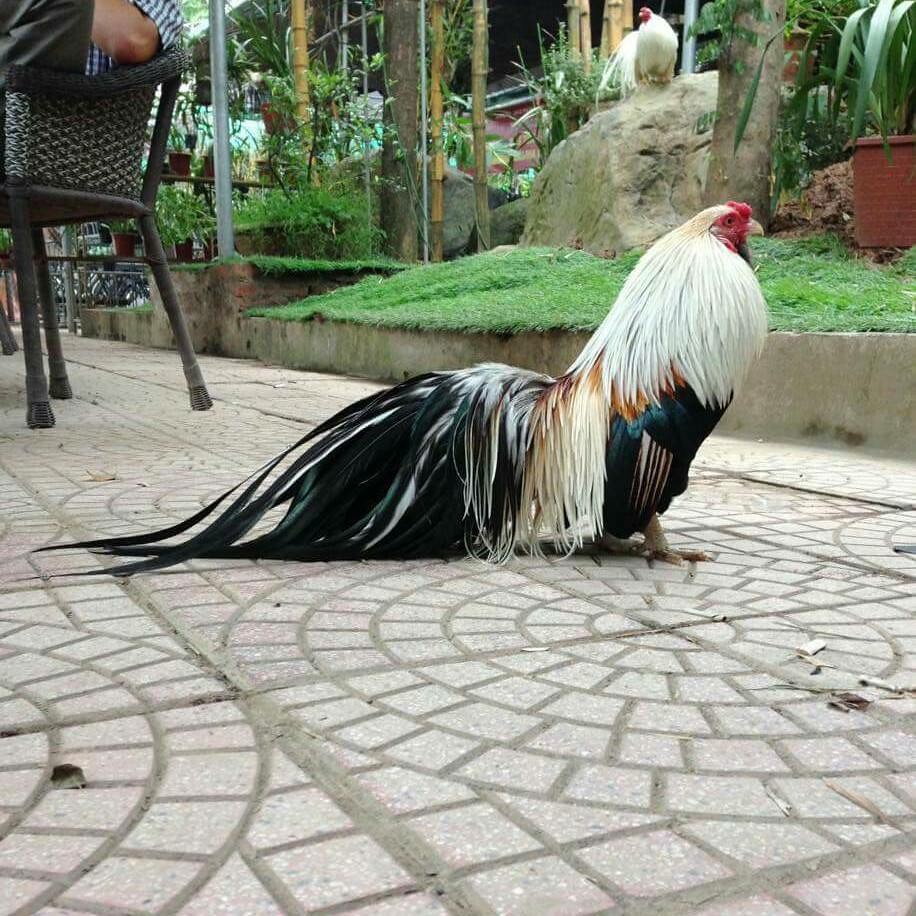In this square-shaped, outdoor photograph, we see a prominent rooster standing on a patterned, interlocking brick ground, possibly within a zoo or a pavilion-like setting. The rooster in the foreground boasts a striking appearance with a predominantly white chest and head, adorned with a hint of red. Its body feathers showcase a mix of bluish-green, yellow, tan, and more red, while its long, black-and-white tail gracefully trails behind. Behind this rooster, perched on a large rock, is another bird—almost entirely white. The backdrop reveals man-made features including grass, potted plants, large stones, and a hint of a natural habitat with trees. In the top left corner, partially obscured, is a rattan patio chair with a gentleman wearing a short-sleeved blue and white checked shirt, though the image cuts off, preventing a full view of him.